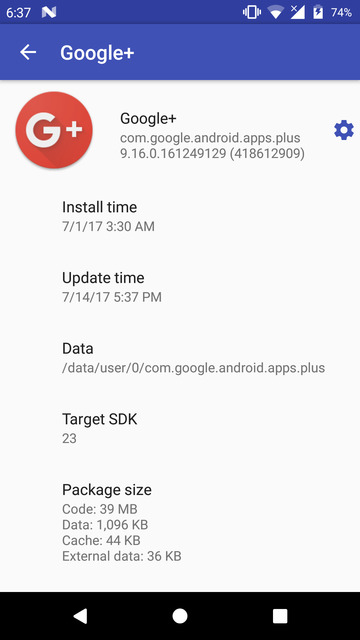The image depicts a screenshot of an Android device, identified by the time displayed as 6:37 in the upper left corner, along with an 'N' icon. Other status icons visible include a vibration icon, Wi-Fi signal, cell signal, and a battery icon indicating a 74% charge.

Below this status bar, a blue banner at the top of the screen reads "Google Plus" alongside a back button. Beneath the banner, there is a prominent red Google Plus button next to text that reads "googleplus.com" and "google.android.apps.plus," followed by a small blue gear icon. Additional details include the installation and update timestamps: installation on 7-1-17 at 3:30am and update on 7-14-17 at 5:37pm.

The section labeled "data" provides further specifics:
- User path: data.user.zero.com.google.android.apps.plus
- Target SDK: 23
- Package size details: 39 MB of code, 1000 KB of data, 44 KB of cache, and 36 KB of external data.

The application interface is primarily white with a blue bar at the top. At the bottom, a black bar houses three navigation icons: a back button, a home button, and a square button for recent apps.